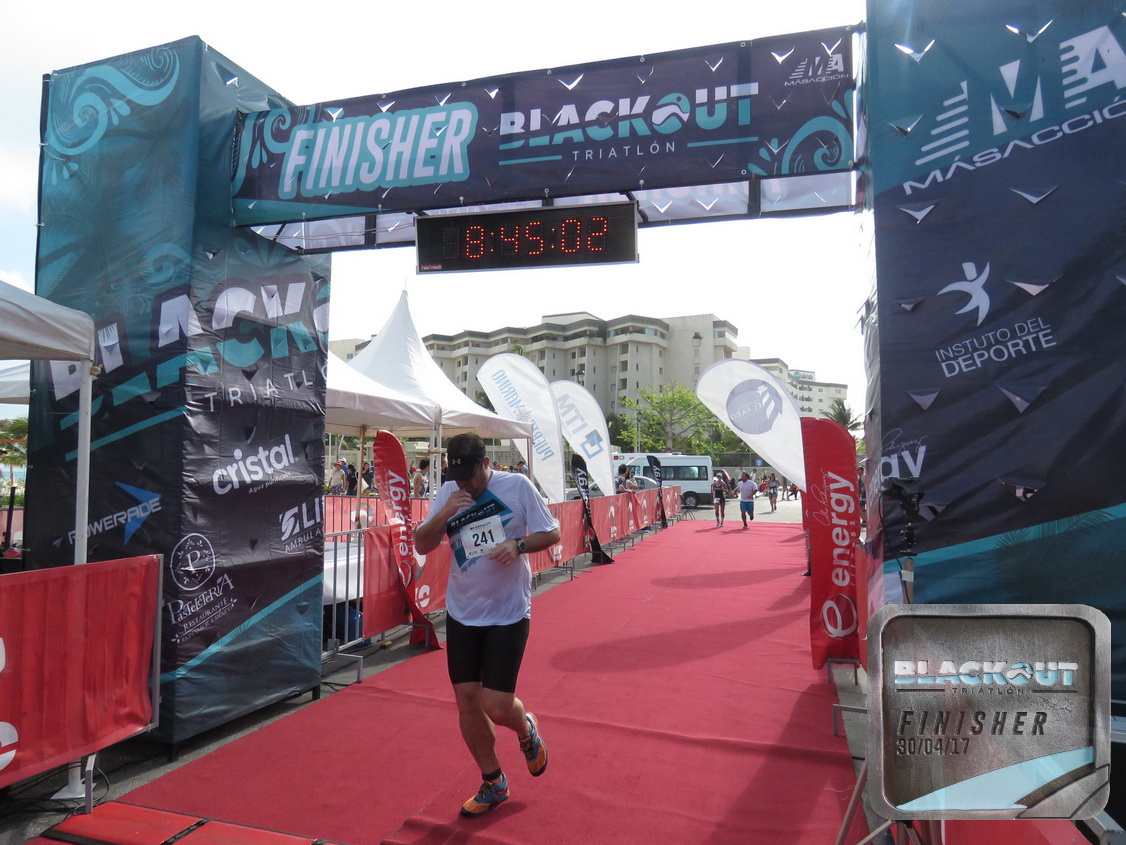The image captures the moment a runner crosses the finish line of a triathlon race. The finish line banner, predominantly colored in shades of blue, prominently displays "Blackout Triathlon" with various sponsor logos including "Crystal Instituto del Deporte Masaccio" and "Energy" on the side columns. The timer above the banner reads 8 hours, 45 minutes, and 2 seconds. The runner, wearing a black cap, a white t-shirt with a blue pattern on the chest, black shorts or pants, and orange shoes, bears the race number 241. He looks downward as he steps onto a green carpet laid at the finish line. Behind him, several other runners are nearing the finish. The background features white tents, red sponsor signs, a building, and a white sky, creating a colorful and busy race scene. The bottom right of the image shows a "Blackout Finisher" date marked as 30/04/17.